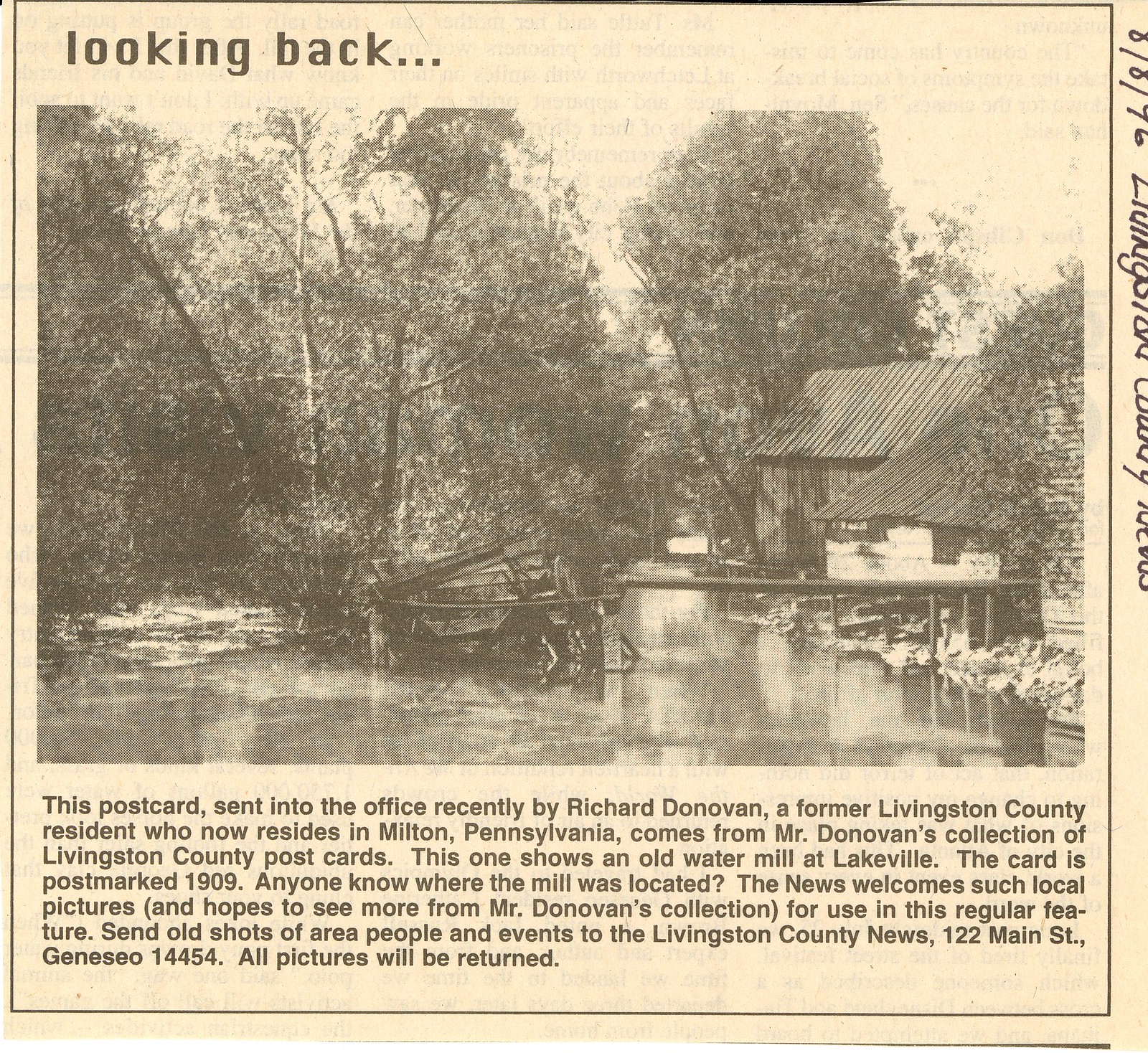The newspaper clipping, tinted in a yellowish hue and showing signs of age, prominently features the segment title "Looking Back" in black font at the top left corner. Below this heading, there is a black-and-white photograph of a serene, wooded area featuring a picturesque river in the foreground. Adjacent to the river stand two wooden structures, likely an old house or barn, both with metal roofs, adding to the rustic charm of the scene. Notably, the building on the right bears the number 8876, accompanied by an indecipherable inscription.

This photograph is revealed to be a postcard, recently submitted to the office by Richard Donovan, a former Livingston County resident who now lives in Milton, Pennsylvania. The postcard is a part of Mr. Donovan's extensive collection of Livingston County memorabilia and dates back to 1909. It depicts an old water mill in Lakeville, sparking a query to the local community about the mill's precise former location.

The accompanying text invites readers to contribute similar historical photos of local people and events. Interested parties are encouraged to send their submissions to the Livingston County News at 122 Main Street, Geneseo, 14454, with the reassurance that all photographs will be returned.